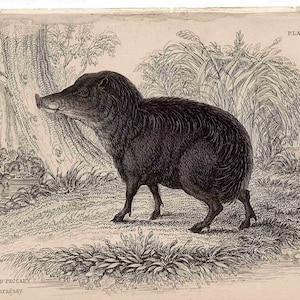This is a very small, detailed black and white drawing of an animal that closely resembles a javelina or boar, situated in a sepia-toned forest background. The animal features a large, hairy body, four thin, hoofed legs, and a pointed snout directed to the left. Its coarse hair runs along its spine, drooping down its sides. The ground beneath its feet appears bare, dotted with grass. Behind the animal, a wide tree trunk stands prominently to the left, accompanied by bushes at its base. On the right, another tree extends its branches like a willow, creating a natural archway over the landscape. The scene is reminiscent of illustrations found in Victorian-era natural history books, combining an intricate depiction of the creature with a minimalist representation of its natural habitat.